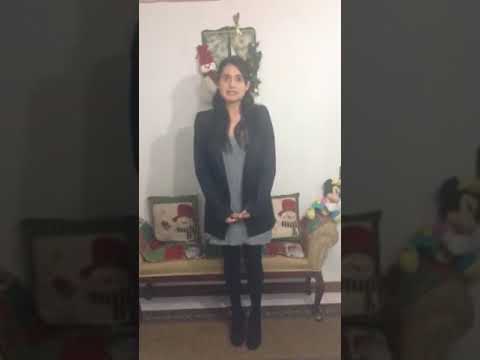The photograph showcases a young woman, approximately 14 to 16 years old, standing at the center. She has olive skin and black hair that cascades past her shoulders. Her attire consists of a black or dark gray blazer, a light gray or green dress underneath, black leggings, and black shoes. She stands on a brown rug, facing the viewer with her eyes closed, seemingly caught mid-blink, and her hands clenched at her sides.

Behind her, a cozy indoor setting is decorated for winter. A small couch with wooden legs, likely light brown or cream in color, is adorned with red, green, and cream decorative pillows featuring snowmen. Next to the couch, a partially visible Minnie Mouse toy peeks from the right edge of the frame. The background also includes a covered bench with two snowman pillows, and a wall with off-white wallpaper that hosts a snowman-themed decoration. The woman's shadow is cast to the left, adding depth to the scene. The photograph, likely taken with a camera phone, is in portrait orientation, with black bars framing the image on either side.